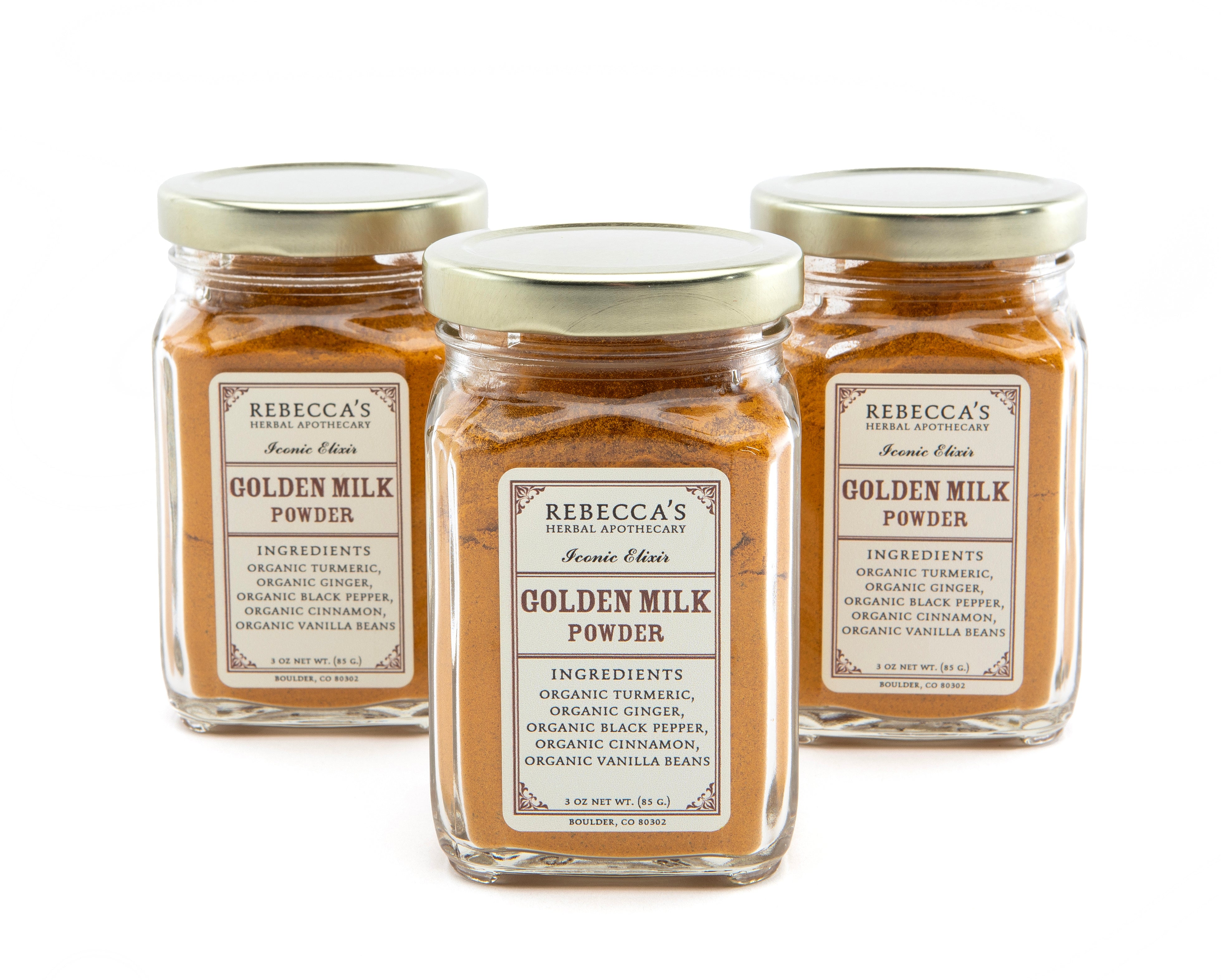The image is a horizontal shot featuring three clear, square-shaped jars of golden milk powder from Rebecca's Herbal Apothecary. Each jar is topped with a gold metal lid and adorned with a white, rectangular label. Positioned in the foreground, one jar sits prominently in front of the other two. The label, which is consistently applied to all jars, reads "Rebecca's Herbal Apothecary" in black text, followed by "Golden Milk Powder" in a brownish-gold font that matches the orangey-brown, almost gold hue of the powder inside. Beneath the product name, the label lists the organic ingredients: turmeric, ginger, black pepper, cinnamon, and vanilla beans, all aligned vertically. The uniformity and detail of the jars emphasize their identical contents and purpose.